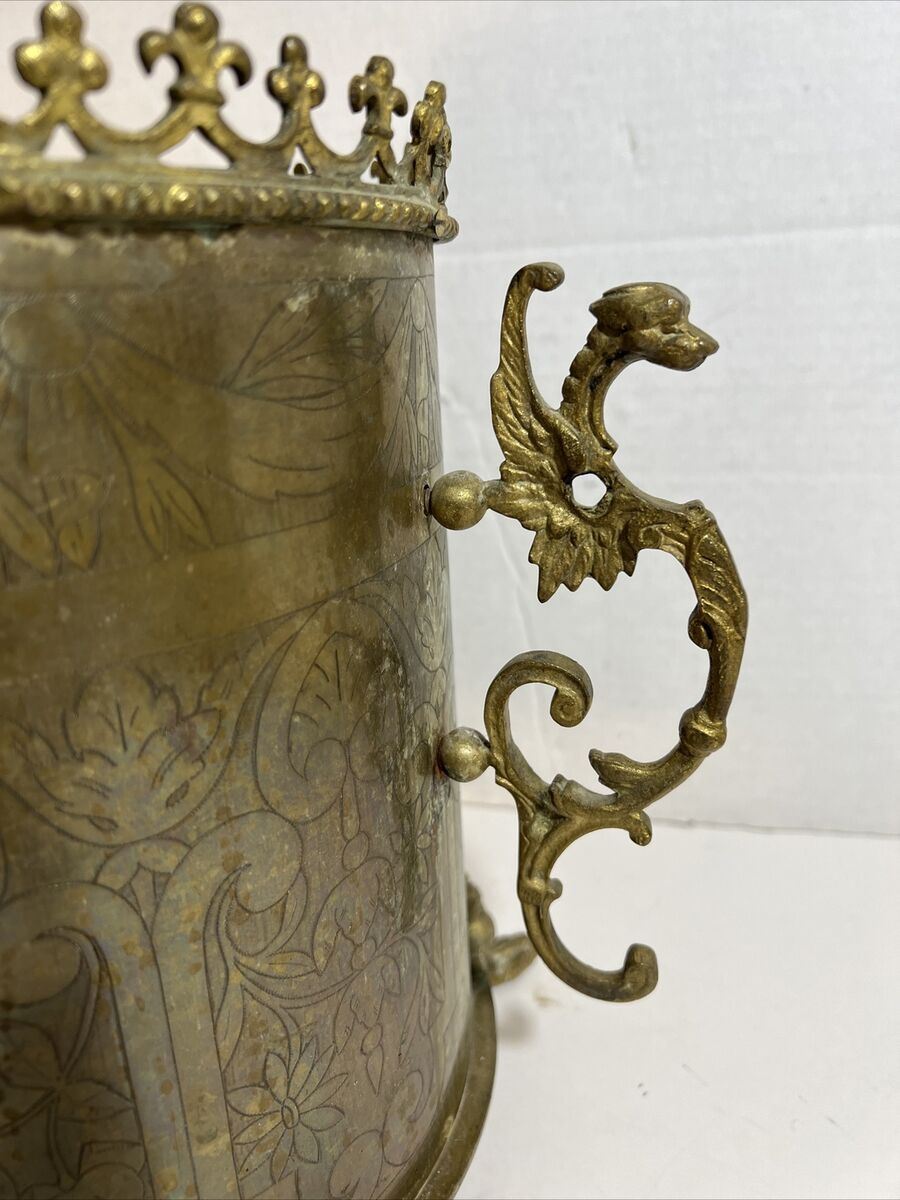The image features an antique, cylindrical brass object that could be a stein or perhaps a decorative crown-like piece. The object appears to be painted gold, giving it a worn, metallic look rather than a genuine golden finish. Only a portion of the item is visible, showing detailed etchings around its surface. The top is adorned with finials reminiscent of fleur-de-lis, and there are various symbols encircling it. Attached to the right-hand side is a thin handle shaped like a dragon, with its wings extending down its body and ending in a curlicue. The dragon's head protrudes outward, as if watching over the piece. The object is placed on a white tiled floor against a tile wall.